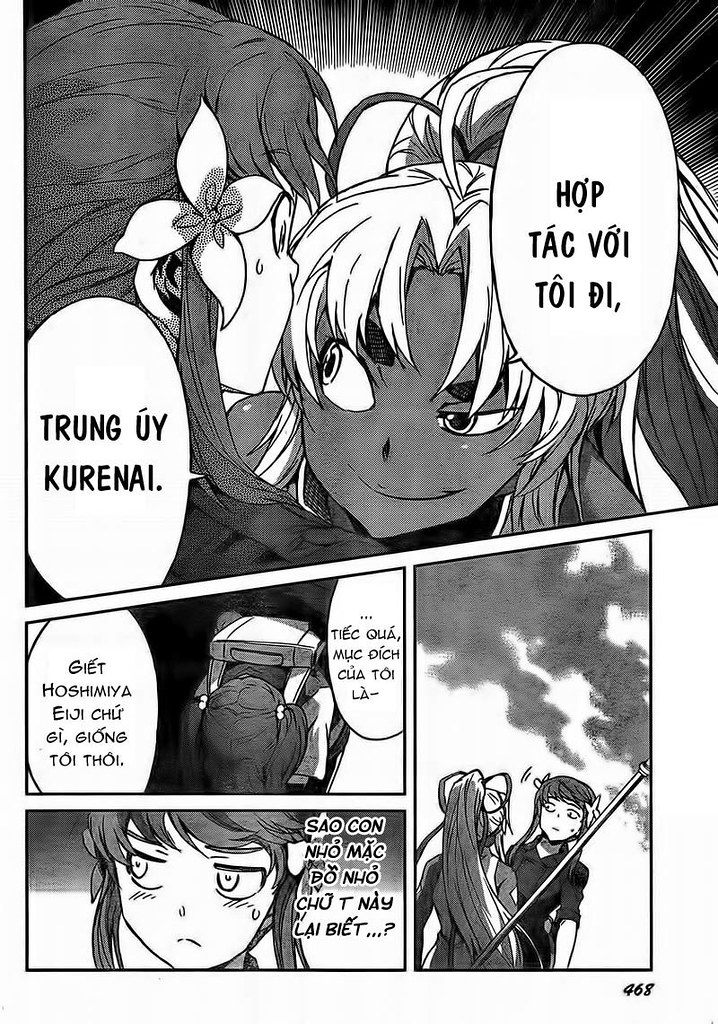This detailed black-and-white image captures a dynamic page from a manga comic book, divided into four distinct panels. The top half is dominated by a large panel showcasing two female characters. The first is a woman with dark skin and flowing white hair, who gazes intently at the second woman— a brunette with fair skin and a flower delicately tucked behind her ear. The brunette has a cynical expression, looking upward from beneath her brow. Speech bubbles in Vietnamese text—reading "TRUNG YAI KURANIYA" and "HOP TAC VOI TOI DI"— suggest a tense conversation.

The remaining three panels are positioned below, each providing further narrative snippets. The first of these supplementary panels is indistinct but implies a transition. The second panel on the bottom left features a close-up of the brunette's face, her expression now shifting to one of distress. In the final panel on the bottom right, the two women are seen from a distance. Here, the brunette, now identified with dark hair, peeks cautiously around the white-haired woman, as if apprehensive about an impending conflict. The intricate artwork and expressive character designs create an engaging visual story, underscored by the mysterious, foreign text.